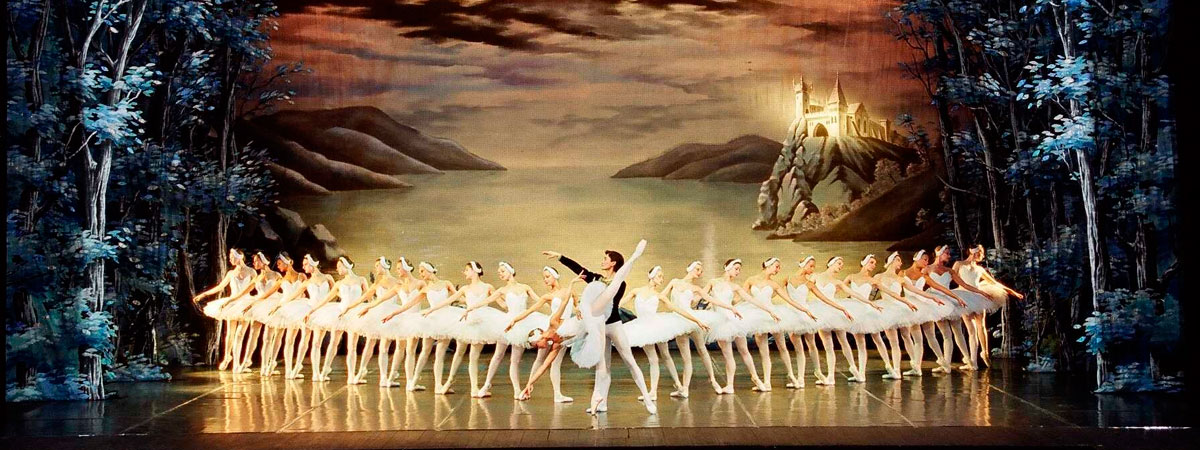The image captures a vibrant stage performance featuring several dancers, including one male and numerous ballerinas lined up gracefully. Dominating the center-left, a performer stands out in a black top and white pants, adding contrast to the composition. The backdrop is a detailed artwork showcasing a serene body of water flanked by towering mountains, adorned with a castle or church on the right side, illuminated by the sun. On either side of the stage, the backdrop also features striking trees with blue leaves, contributing to the overall ethereal atmosphere. The scene is rich with colors like white, blue, brown, gray, black, tan, and red, enhancing the visual beauty and depth of the theatrical performance.